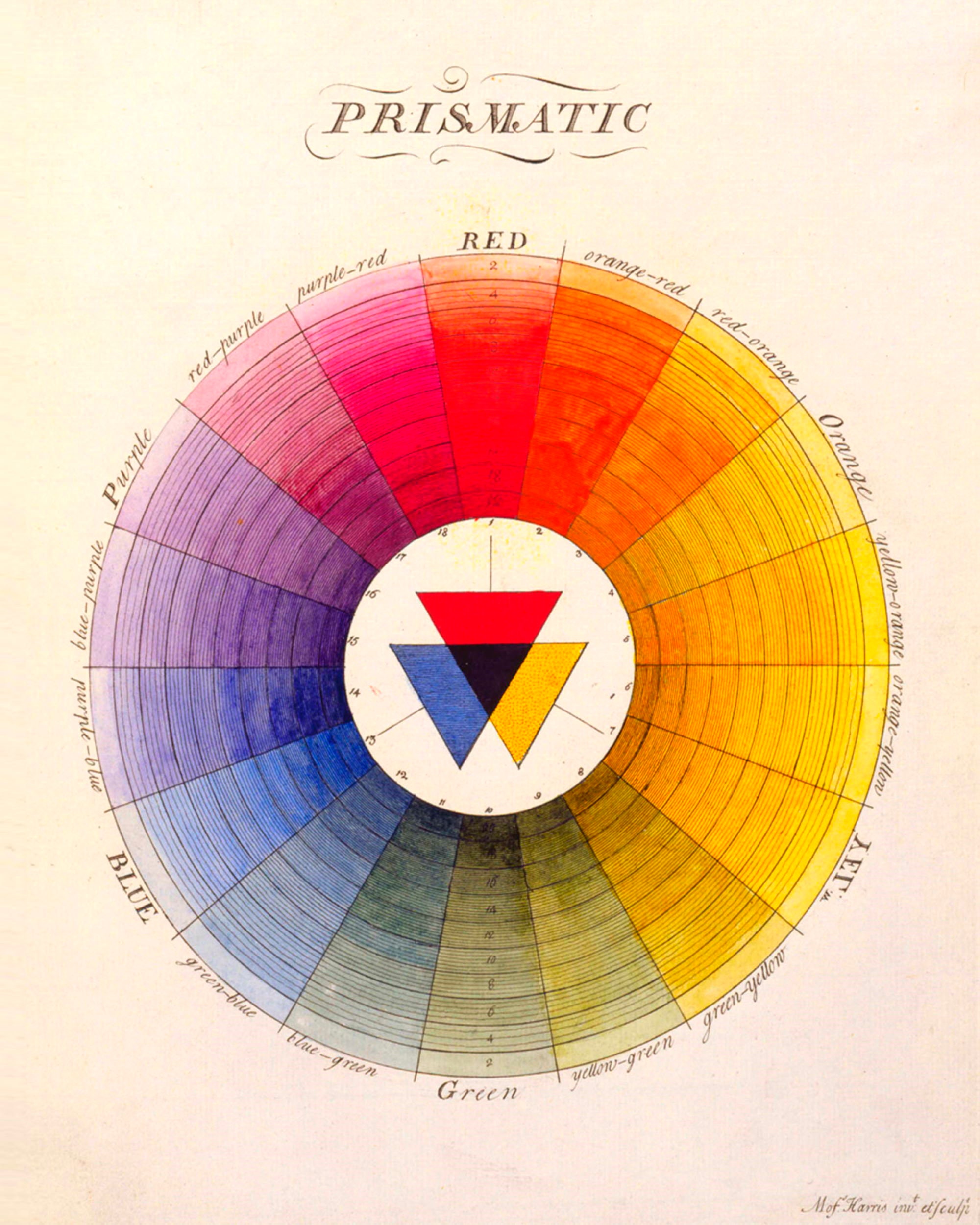The image depicts a detailed color wheel artwork set against a subtly toned background that transitions from a yellowish hue in the upper left to a more tannish overall shade. The color wheel itself is a large, circular design split into pie-shaped segments, each labeled with colors progressing in a spectrum: starting from "red" at the top and moving through "red-orange," "orange," "yellow-orange," "yellow," "yellow-green," "green," "blue-green," "blue," "blue-purple," "purple," "red-purple," and back to "red" again. Each segment showcases gradients of the respective color, transitioning from lighter shades on the outer edge to darker shades towards the center.

Encircling the vibrant spectrum is an interior white circle where three downward-pointing triangles intersect, forming a central black triangle where their tips meet. The triangles are distinctly colored: the left one is blue, the top one is red, and the right one is mustard yellow. Above the wheel, the word "Prismatic" is inscribed in black, while the bottom right corner bears initials in a foreign language. Numbers encircle the wheel, numbering 1 through 18 in a counterclockwise direction. Additionally, words around the circle appear to provide inspirational themes related to the colors displayed.